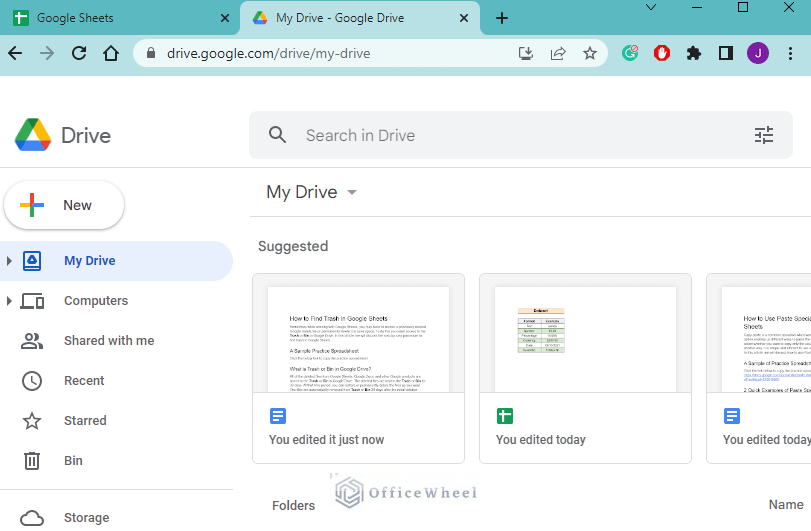In this image, a browser window is visible, with multiple tabs open. On the left, there's a tab for Google Sheets, marked by a small green icon with a white cross. The highlighted tab next to it is titled "My Drive - Google Drive." Below the tabs, the URL bar displays "drive.google.com/drive/my-drive," accompanied by various browser icons and several extensions in the top right corner.

The content within the browser window shows the Google Drive interface. At the upper left, "Drive" is prominently displayed. Beneath it, the "New" button is visible, followed by "My Drive" highlighted in blue. Along the left side of the screen, a sidebar lists navigational options: Computers, Shared with Me, Recent, Starred, Bin, and Storage.

To the right of the sidebar, a search bar labeled "Search in Drive" is prominently placed. Just below this bar are labels: My Drive (with a downward arrow indicating a dropdown menu) and Suggested. The central part of the screen displays three boxes, each representing different documents. The first box states "You edited just now," indicating a recently edited document. The second and third boxes both say "You edited today," showing a chart and another document, respectively.

Below these document previews, the "Folders" section is visible, with a folder named "Office Wheel." At the bottom right of the screen, the label "Name" is located, suggesting sorting options for the files and folders. The overall image provides a detailed snapshot of the Google Drive user interface, highlighting recent activity and navigation features.